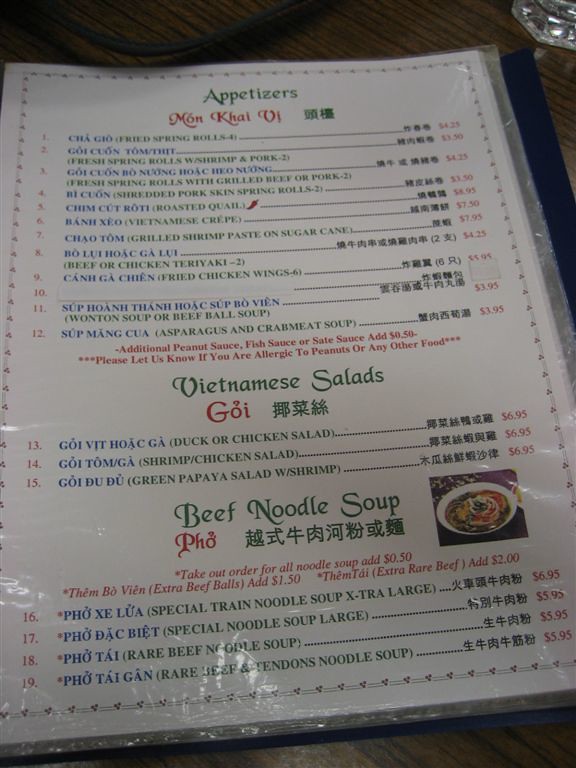This image captures a diverse and colorful menu from a Vietnamese or Chinese restaurant. The menu is presented on a white sheet of paper, bordered by a pattern of three dots followed by a line. The text is in multiple colors and languages: blue for Vietnamese, green for English, black for Chinese, and red for the prices.

Starting from the top, the menu lists the appetizers:

- Fried Spring Rolls (4 pieces) - $4.25
- Fresh Spring Rolls with Shrimp and Pork (2 pieces) - $3.50
- Fresh Spring Rolls with Grilled Beef or Pork (2 pieces) - $4.25
- Shredded Pork Skin Spring Rolls (2 pieces) - $3.50
- Roasted Quail (marked as spicy) - $8.95
- Vietnamese Crepe - $7.50
- Grilled Shrimp Paste on Sugar Cane - $7.95
- Beef or Chicken Teriyaki (2 pieces) - $4.25
- Fried Chicken Wings (6 pieces) - $5.95
- Wonton Soup or Beef Ball Soup - $3.95
- Asparagus and Crab Meat Soup - $3.95

Next, a note in red indicates additional charges for sauces: peanut sauce, fish sauce, or sauté sauce for an extra $0.50. The menu also advises customers to inform the staff of any peanut or other food allergies.

The following section features Vietnamese salads:

- Duck or Chicken Salad - $6.95
- Shrimp and Chicken Salad - $6.95
- Green Papaya Salad with Shrimp - $6.95

The last section is dedicated to beef noodle soup or pho options:

- Special Trained Noodle Soup (Extra Large) - $6.95
- Special Noodle Soup (Large) - $5.95
- Rare Beef Noodle Soup - $5.95
- Rare Beef and Tendon Noodle Soup - $5.95

Under the beef noodle soup section, there are additional takeout options and extras:

- Take-out order for all noodle soups - Extra $0.50
- Extra Beef Balls - $1.50
- Extra Rare Beef - $2.00